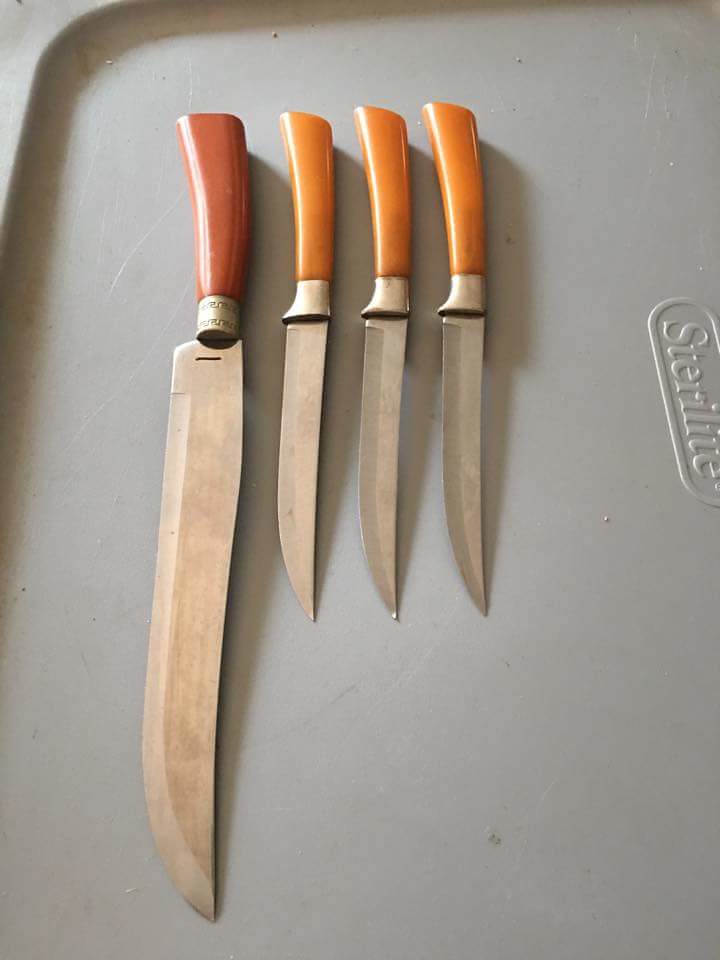The image displays a top-down view of four knives neatly arranged on a gray Sterilite plastic tub lid. The lid serves as a clean and simple background, emphasizing the details of the knives. The handles of the knives, oriented upwards, appear carved and are a golden orangish color, possibly made of bone or wood, with the leftmost knife having a slightly darker handle. The blades are silver and shiny, with the edges curving to form a more narrow and softer point than usual. The knife on the far left is notably longer and thicker, likely intended for chopping, while the other three knives are shorter and identical, suitable for use as steak or paring knives. The stark contrast between the knives' meticulous craftsmanship and the plain, utilitarian plastic lid highlights their intricate design and functional beauty.